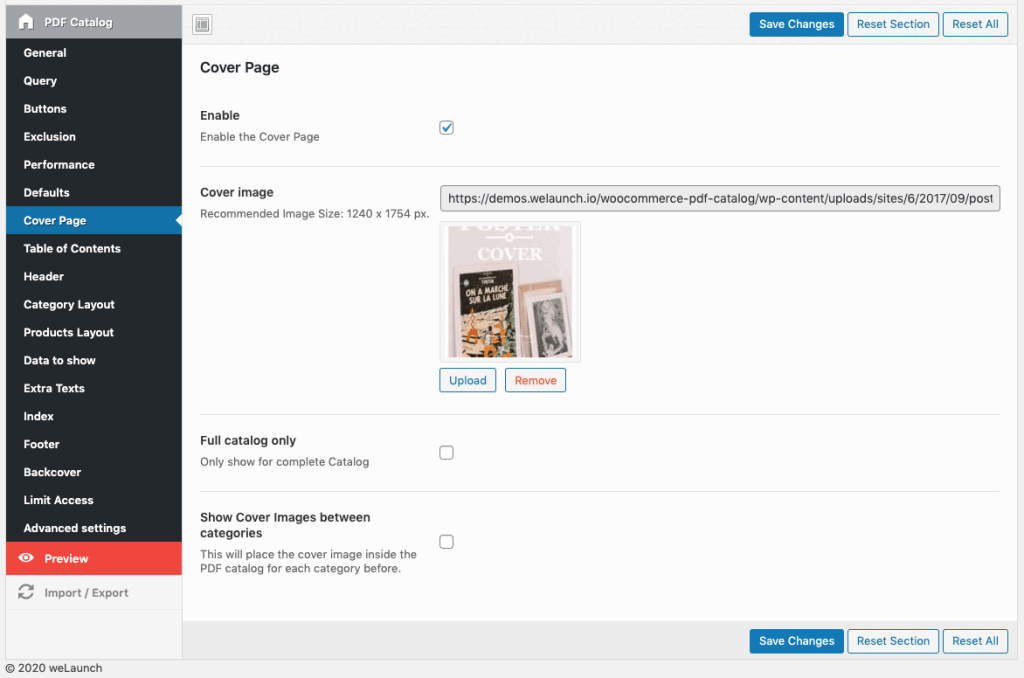The image displays a detailed view of a webpage interface designed for managing a PDF catalog. 

**Top Section:**
- On the top left, there is a label "PDF Catalog" accompanied by a house icon, both in white set against a dark gray bezel.
- On the top right, within a medium gray bezel, there is a square icon resembling a newspaper in gray. 

**Button Section:**
- To the right, a dark blue button with white text reads "Save Changes."
- Adjacent to this are two more buttons:
  - One with a blue border and blue text that reads "Reset Section."
  - Another with a blue border and blue text that reads "Reset All." 

**Sidebar (Left-Hand Side):**
- The left sidebar is a dark black rectangle with multiple cascading selections, labeled as follows:
  - General
  - Query
  - Buttons
  - Exclusion
  - Performance
  - Defaults
  - **Cover Page** (highlighted in dark blue with a white arrow indicating it is selected)
  - Table of Contents
  - Header
  - Category Layout
  - Products Layout
  - Data to Show
  - Extra Text
  - Index
  - Footer
  - Back Cover
  - Limited Access
  - Advanced Settings
- Another section highlighted in orange features an eyeball icon with "Preview" labeled to the left. 
- Below this, there is a refresh symbol followed by "Import/Export."

**Main Content Area:**
- The primary section is labeled "Cover Page" with "Enable" in bold black text directly below.
- In gray text, it reads "Enable the Cover Page" alongside a checked green box.
- Below this is a section titled "Cover Image" with a long address on the right.
- There is also a note stating "Recommended Image Size 1240 x 1756 pixels."
- An image of books is displayed with a background captioned "Cover" in pink.
- Underneath, there is an option labeled "Full Catalog Only" with a corresponding unchecked box and a note in gray that says "Only Show for Complete Catalog."
- A subsequent option states "Show Cover Images Between Catalogs," followed by a gray note explaining that this setting will place the cover image inside the PDF catalog for each category before.

**Bottom Buttons:**
- At the bottom, three buttons are present:
  - A dark blue button with white text stating "Save Changes."
  - A white button with a blue border and blue text reading "Reset Selection."
  - Another similar button labeled "Reset All."

This detailed description captures every element and visual cue presented on the webpage interface for managing the PDF catalog.